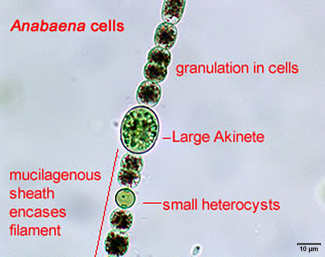The microscope photograph, framed in a perfect square, showcases a detailed strand of anabaena cells. The strand, with its cells appearing in a diagonal line from the top center to the bottom center, is set against a blurry gray background peppered with out-of-focus circles. The anabaena cells, encased in a mucilaginous sheath, are small ringed circles containing dark green and light green dots. Red text overlays the image, providing key annotations: "anabena cells" is noted at the top left, "granulation in cells" appears to the right of the line of cells, "large akinete" marks a prominent larger green cell near the center, and "small heterocysts" identifies a smaller cell below it. Additionally, at the bottom left, "mucilaginous sheath encased filament" is labeled. A measurement key in the bottom right corner specifies "10 µm," offering a scale for understanding the cell sizes. Overall, the image presents a close-up view of these intricately detailed, science-rich cellular structures.